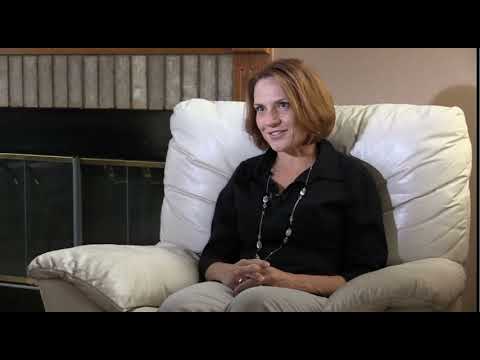In the photograph, five women stand closely together, holding up a bright yellow sign that reads "Global Walk." The poster features a picture of the earth against a dark blue background, adorned with a moon and stars, and includes a blue and gold lion's logo at the bottom. The group predominantly consists of Middle Eastern women wearing vibrant, diverse outfits. On the left, a woman in a white dress with a black stripe over her chest, black hair, and a gold bracelet stands confidently. Next to her, a darker-skinned woman in a black dress and glasses holds the sign with one hand. At the center, a Caucasian woman in a white suit with a yellow headband smiles broadly, revealing her top row of teeth. To her right, a woman in a pink dress with a black wristwatch appears somewhat anxious. The furthest on the right is an overweight woman in a black shirt, frowning slightly, with a bindi on her forehead. The background shows white walls and ceilings with lights, and on the left side, another man with black hair, glasses, a dark shirt, and white pants is visible. The image is set within a larger black background, adding a framing effect.